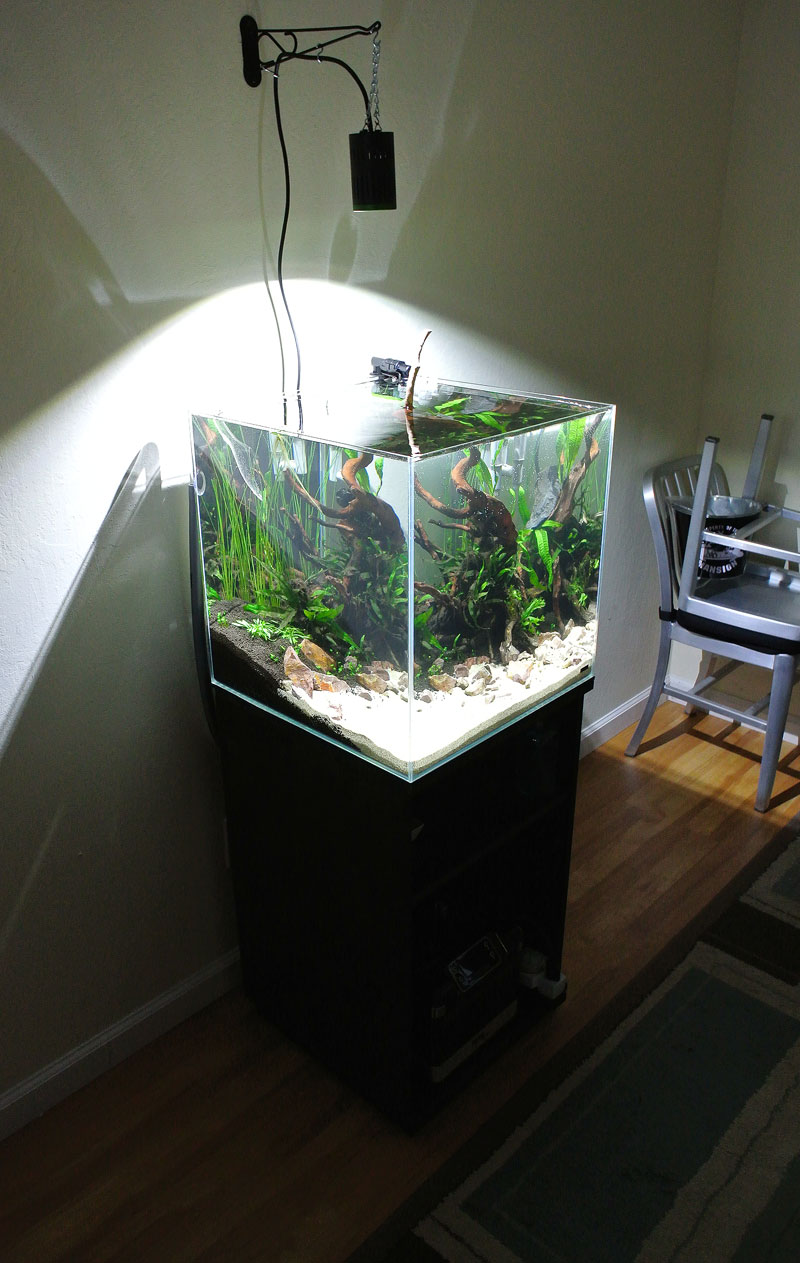This image depicts a beautifully maintained cube-shaped aquarium situated in a darkened room. The aquarium, which measures equal on all sides, rests on a sturdy black rectangular pedestal. Inside the aquarium, intricate elements such as lush greenery, sand, and brown rocks are visible, along with a prominent piece of wood resembling an underwater tree, partly emerging from the top, indicating the absence of a lid. The tank's interior is artfully illuminated by a white light hanging from a hook above, casting a soft glow on the vibrant plant life but revealing no visible aquatic animals. The aquarium is set on a yellow wooden floor adjacent to a notable area rug. In the room's corner stands a silver metal chair with another identical chair balanced on top. The walls behind the setup are painted white, contributing to the serene atmosphere of this meticulously arranged home space.